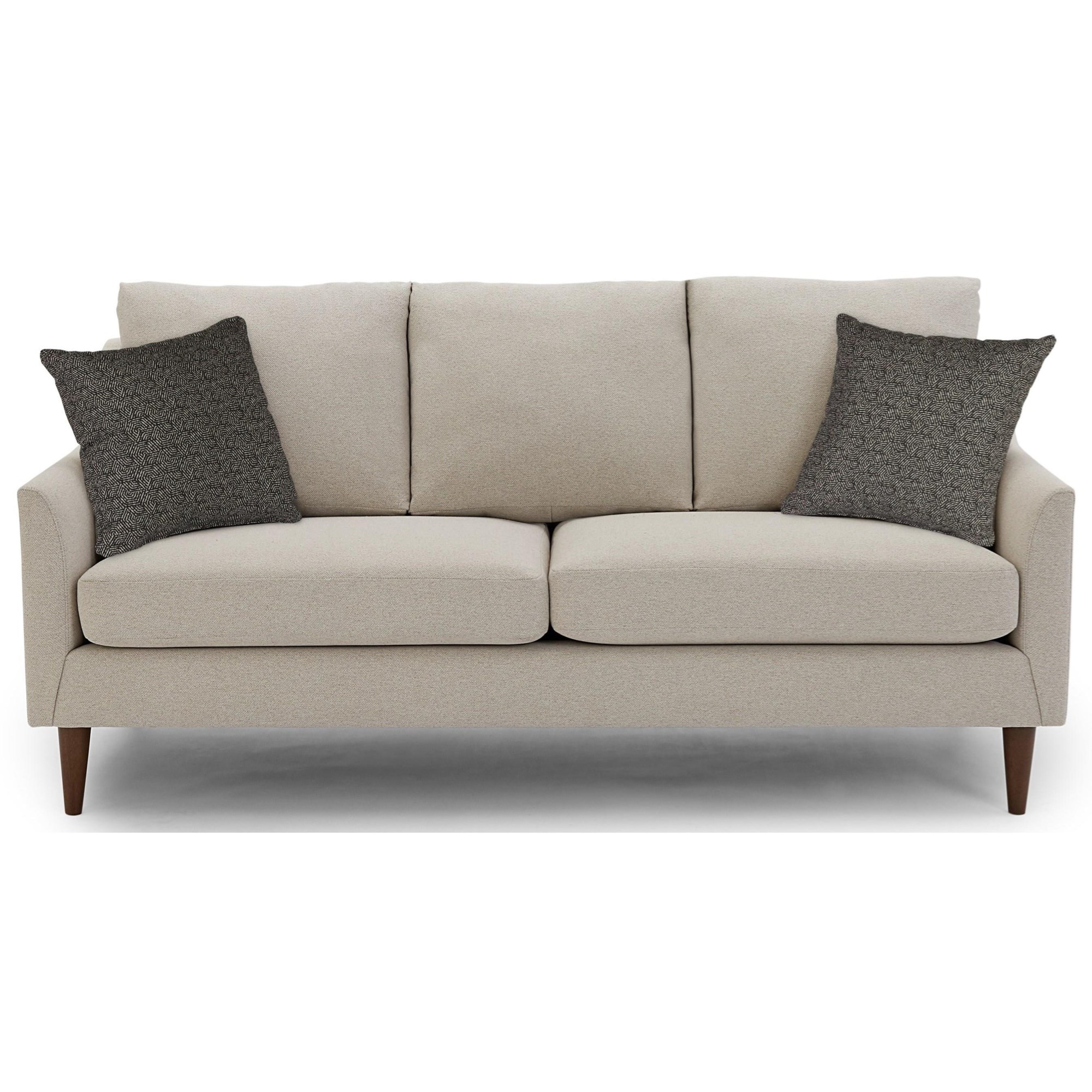This image features a modern, sleek, and symmetrical light grey sofa, set against a plain white background. The couch's design is characterized by its straight, angular lines, with minimal curves and a somewhat stiff appearance. It stands about six inches off the floor on small, dark brown wooden legs, creating an open space underneath. The sofa is structured with two large seat cushions and three sizeable back pillows. On each side of the couch, there are two darker throw pillows with speckles of white, adding a subtle contrast. The armrests appear angular and not particularly cushioned, reflecting the overall modern aesthetic of the piece. The symmetry and clean lines make this piece stylish yet simple, suitable for a contemporary living space.